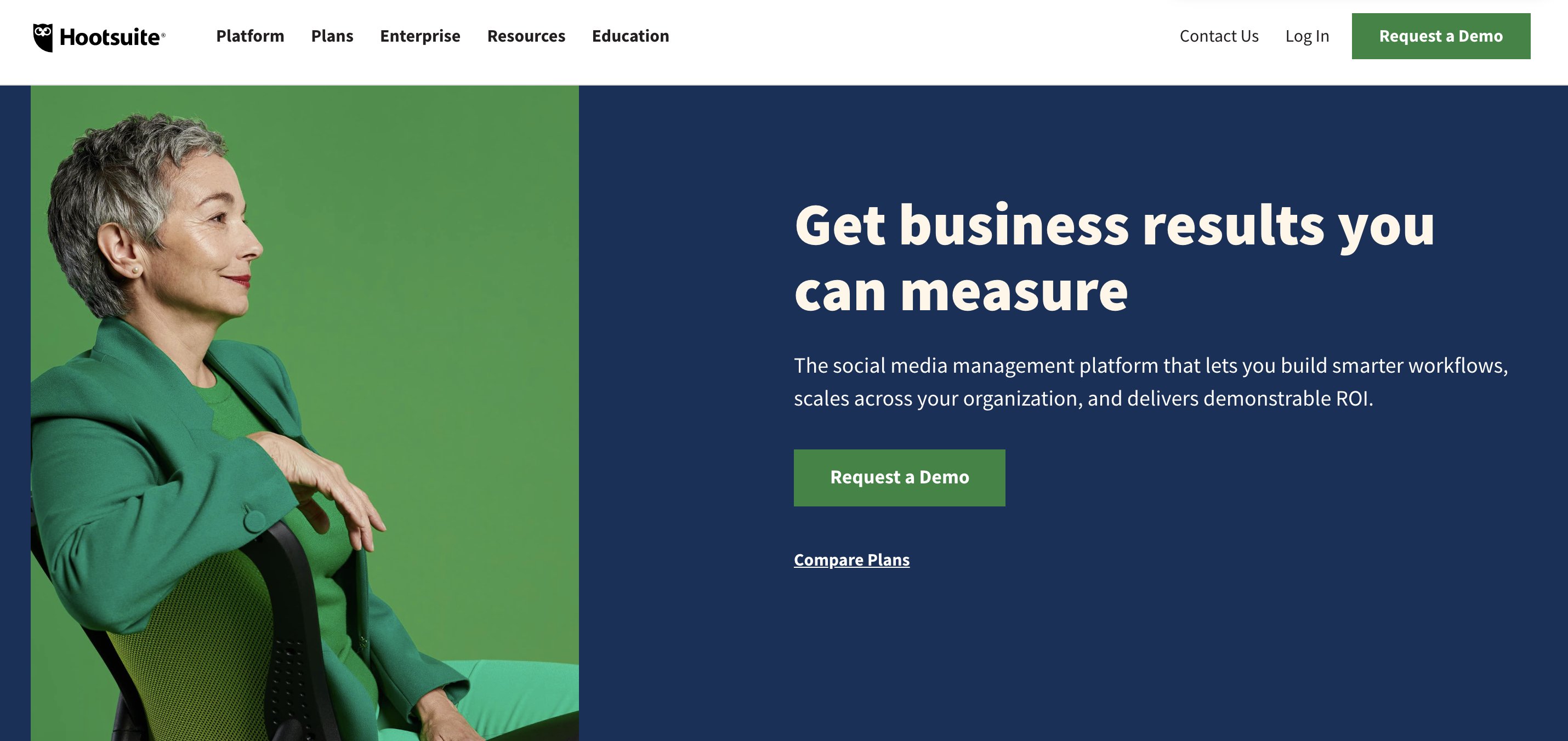This is a screenshot from the HootSuite website. In the upper left-hand corner, the word "HootSuite" is displayed in black font next to a logo of an owl. The logo features just the front of the owl, highlighting its prominent eyes, with the bottom of the logo tapering to a point that curves to the right. 

Immediately to the right of the HootSuite logo, there is a navigation menu with the following options: "Platform," "Plans," "Enterprise," "Resources," and "Education." On the upper right side of the screen, the options "Contact Us," "Log In," and a green button labeled "Request a Demo" in white font are visible. 

In the main content window of the website, a woman wearing a green suit coat is seated on a chair. The back of the chair is angled towards the lower left side of the image. The woman is positioned such that the chair's back is under her right arm.